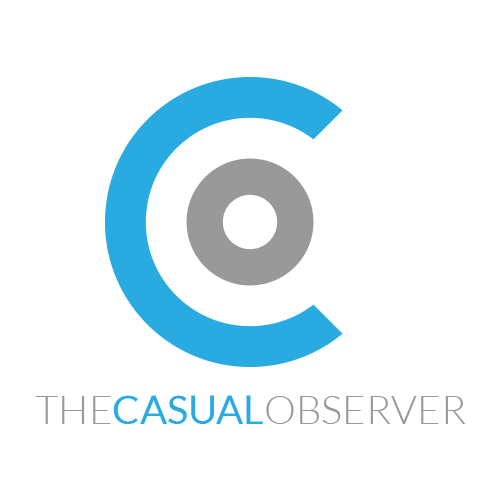The image features a company logo centrally placed on a white background with text below it. The logo comprises a thick, blue, three-quarter circle forming the letter "C", encapsulating a gray donut-shaped circle, which itself has a white center. Beneath this emblem, the text "THECASUALOBSERVER" is written in all capital letters with no spaces between the words. The word "THE" is in gray, "CASUAL" is in light blue, and "OBSERVER" returns to gray, matching the color scheme of the logo. The blue "C" likely represents "Casual," while the gray circle symbolizes "Observer."